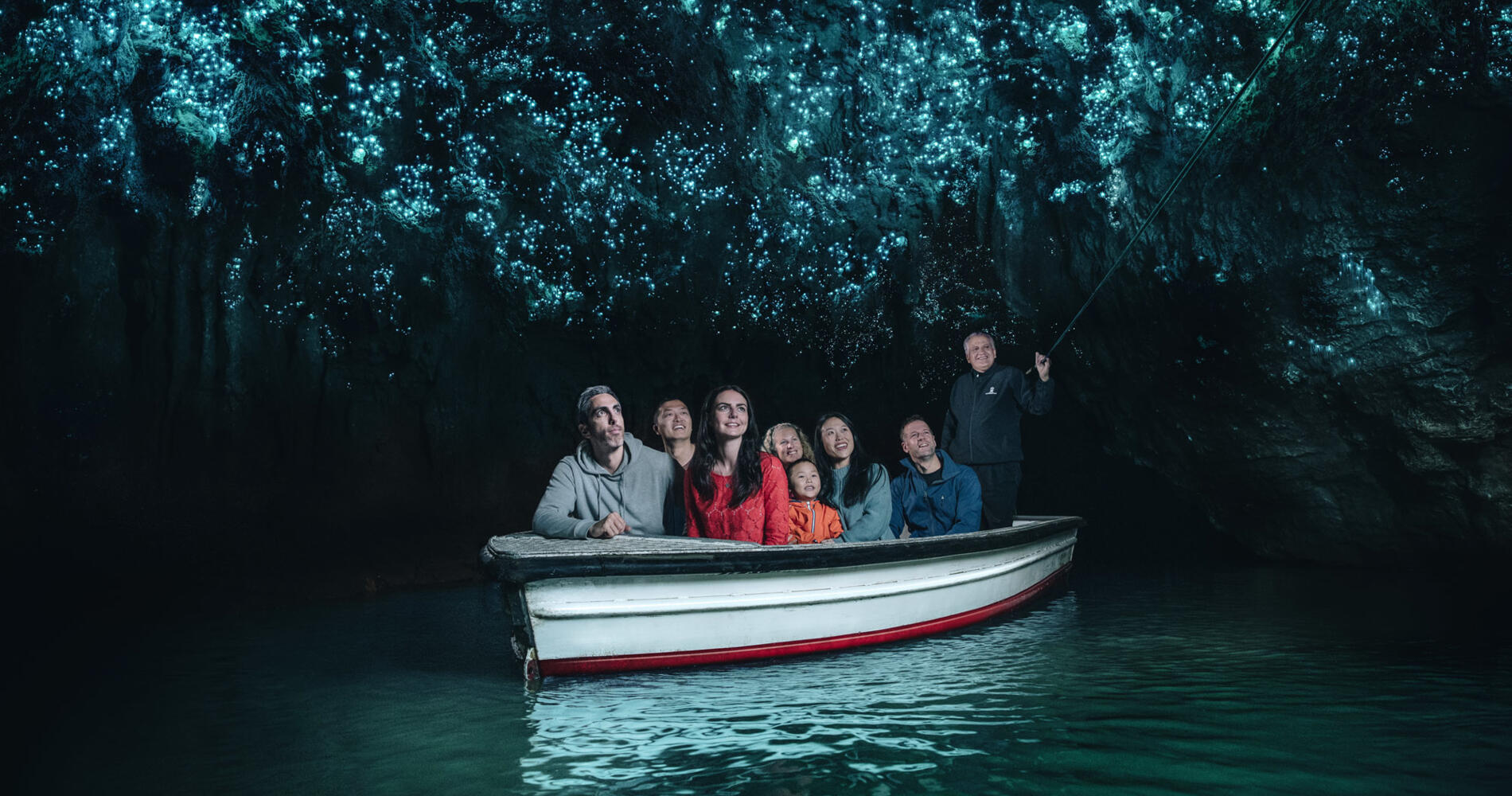This is an intricately detailed night-time photograph that appears to have been heavily photoshopped. The focal point is a small white boat, possibly a canoe or rowboat, floating on eerily still water that has a bluish-gray-green hue with subtle ripples. The scene is enveloped in darkness, with dark trees silhouetted against a cave-like backdrop, punctuated by natural-looking neon blue and green lights that give an otherworldly feel.

Inside the boat are eight people, a mix of adults and children, positioned in a way that makes them appear digitally inserted, as their scale seems improbable for the small vessel. The group includes: a man in a gray sweatshirt at the front, a woman with long brunette hair in a red long-sleeved top next to him, a little Asian girl in an orange top behind her, a blonde woman seated next, the little girl's presumed mother in a long blue-gray shirt to her right, another man in a blue shirt sitting behind her, another seated man behind the man in the gray sweatshirt, and finally, an older man standing at the stern. The older man is holding a laser pointer aloft, directing everyone's gaze upwards as if pointing at something significant—perhaps stars or objects in the cave ceiling, contributing to the surreal atmosphere of the image.